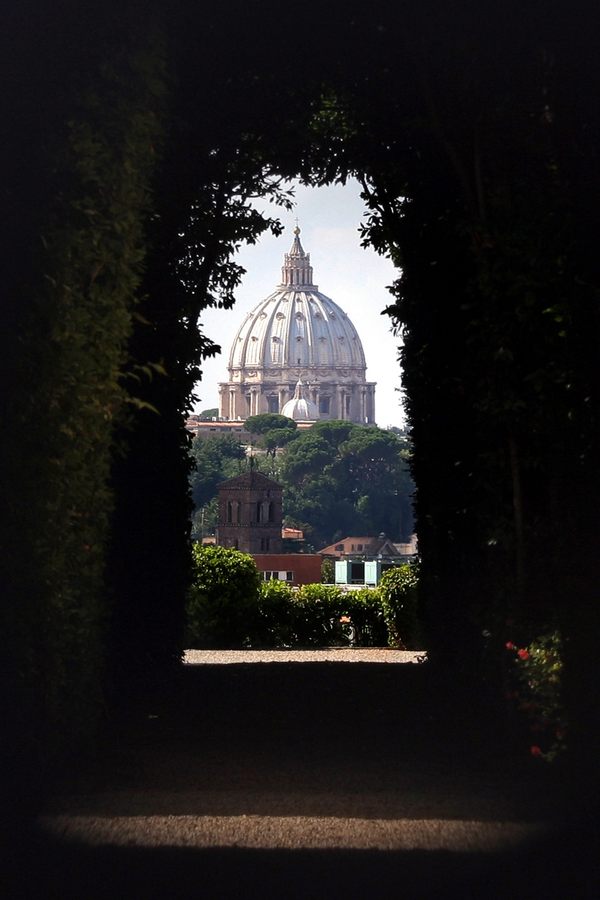The photograph captures an outdoor daytime scene, framed through a dark archway or window covered by tree branches. The arch creates a natural frame, highlighting a sequence of structures in the distance. The immediate foreground features dark gray stone ledges, leading to silhouetted tree branches on either side. Midground reveals green hedges and a lower-level building. Further back, there's a small cupola in front of a larger, more prominent dome topped with a spire and a cross. The sky is a clear blue, contrasting with the dark, shadowed foreground and adding depth to the architectural elements, suggesting the ornate structure might be a grand Capitol building or an elaborate church. The use of the archway and surrounding greenery to frame the distant domes adds a sophisticated, artistic touch to the composition.